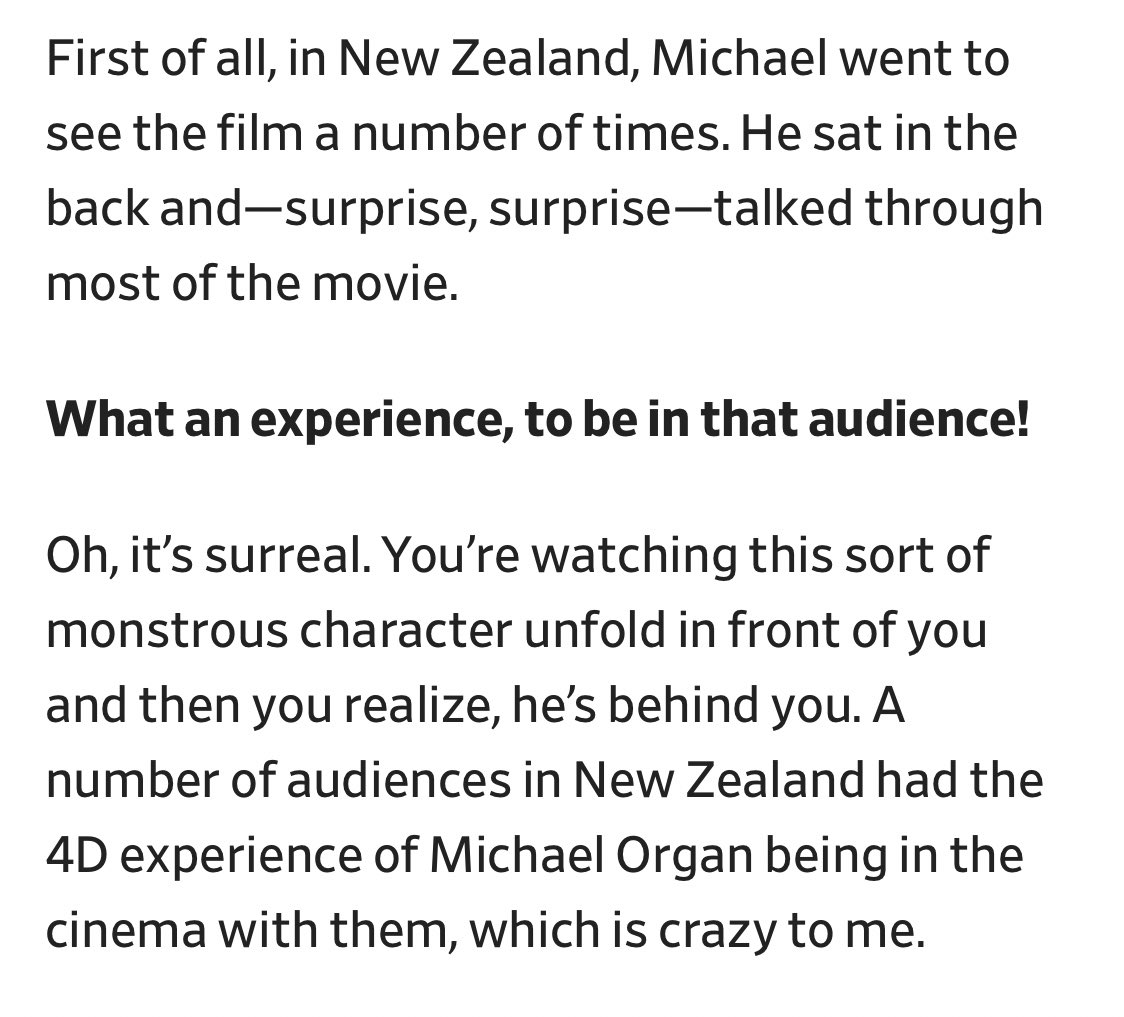The image displays black Times New Roman text on a white background, divided into two regular paragraphs with a single bolded line in between. At the top, it reads, "First of all, in New Zealand, Michael went to see the film a number of times. He sat in the back and, surprise surprise, talked through most of the movie." In the middle, in bold black text, it states, "What an experience to be in that audience." The text then continues, "Oh, it's surreal. You're watching this sort of monstrous character unfold in front of you, and then you realize he's behind you. A number of audiences in New Zealand had the 4D experience of Michael Organ being in the cinema with them, which is crazy to me." The overall layout is simple and clear, resembling something that might be seen in a book or magazine article. The text is perfectly spaced and highly legible against the white background.